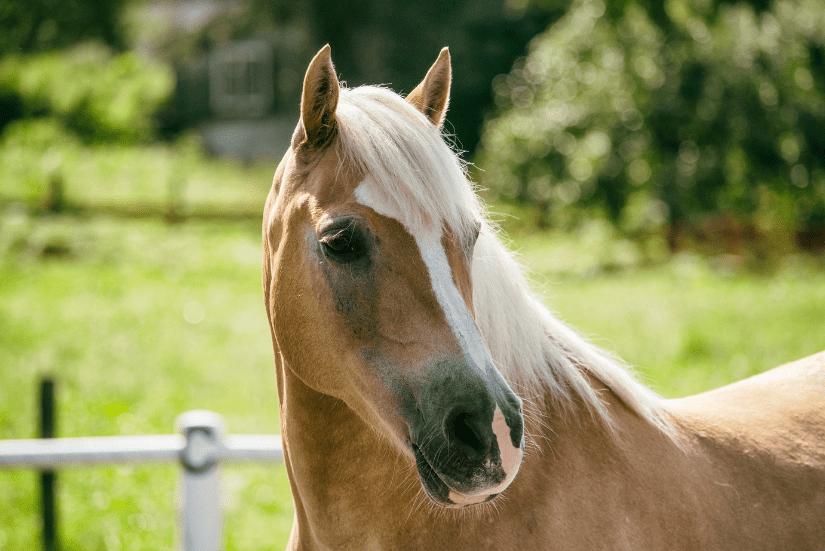The well-lit, outdoor image captures the shoulder-up view of a palomino horse as the main subject, set against a blurred background. The horse, positioned towards the right of the wide vertical shot, has a tan coat with a distinctive large white stripe running down its face to its black snout, which also has pink highlights. Its blonde mane elegantly extends down its neck, and some hair falls between its erect ears, which are attentively pointed in the direction it’s looking. The horse, exuding a muscular and strong presence, appears relaxed with its brown eyes gazing right. Behind the horse, blurred elements include a white metal fence, a distant house, a courtyard with green grass, and trees with lush green leaves, adding depth and context to the serene scene.